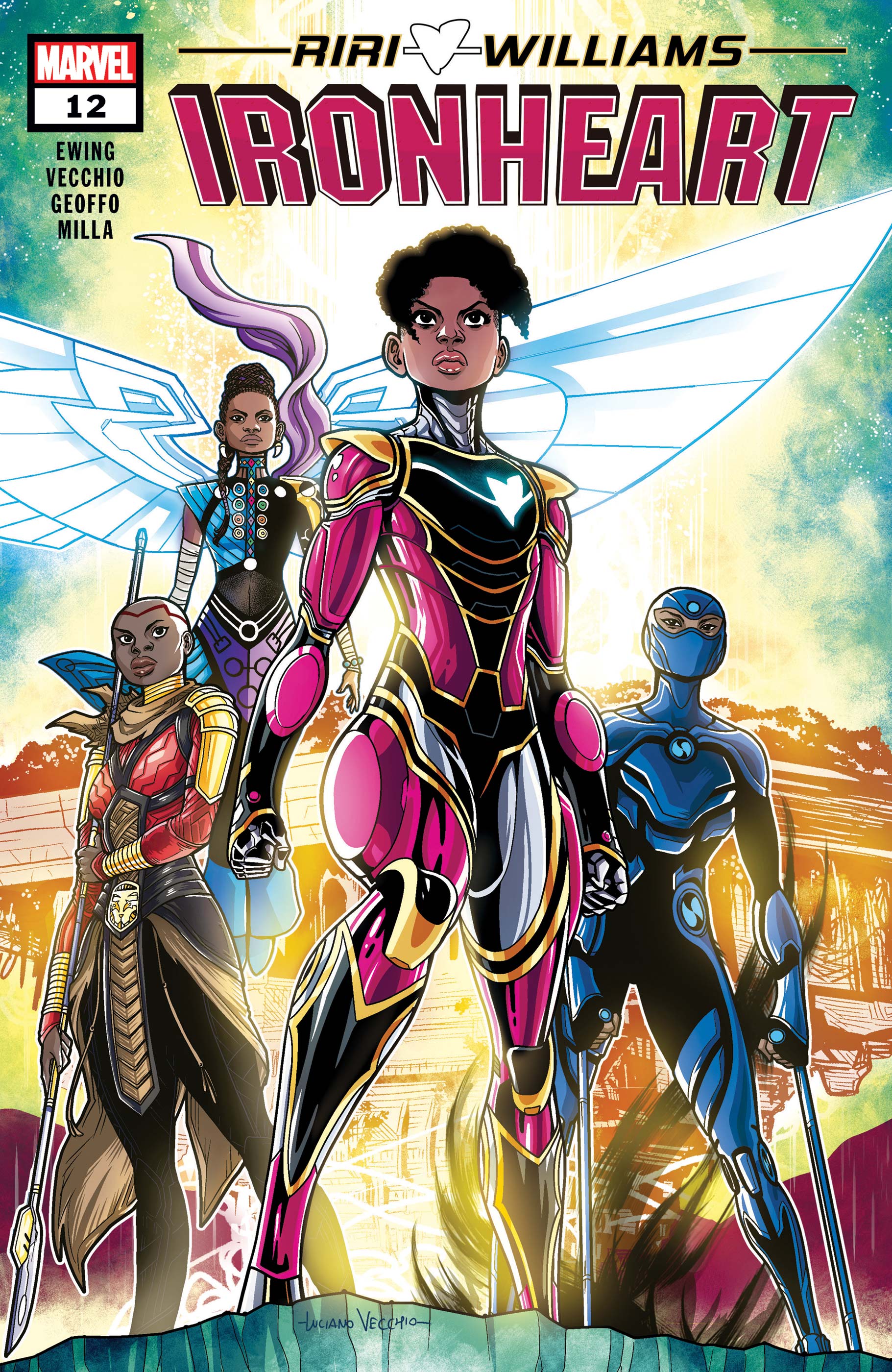This comic book cover titled "Ironheart" prominently features the protagonist Riri Williams, as indicated by the text at the top in red letters with a heart between "Riri" and "Williams." The rectangular image is vertical, with a blocky pink-colored font showcasing the title "Ironheart" beneath it. In the upper left corner, the Marvel logo sits in a red and white square, followed by the number 12, and the names Ewing, Vecchio, Yofo, and Milla in black letters below.

The central heroine, Ironheart, a young black woman, stands triumphantly in a tight-fitting, elaborate mech suit that is primarily black and pink with gold accents. Her suit features a white flower motif over her heart. Flanking her are three other characters: to her right, a ninja-like figure dressed entirely in blue and black; to her left, a female warrior resembling a tribal African fighter, holding a giant pike; and in the background, an angelic figure with cybernetic wings that are white, black, and silver, evoking a sense of future-tech aesthetics. The characters collectively strike a heroic pose, reminiscent of those from a Wakanda Forever-like universe, exuding strength and unity.